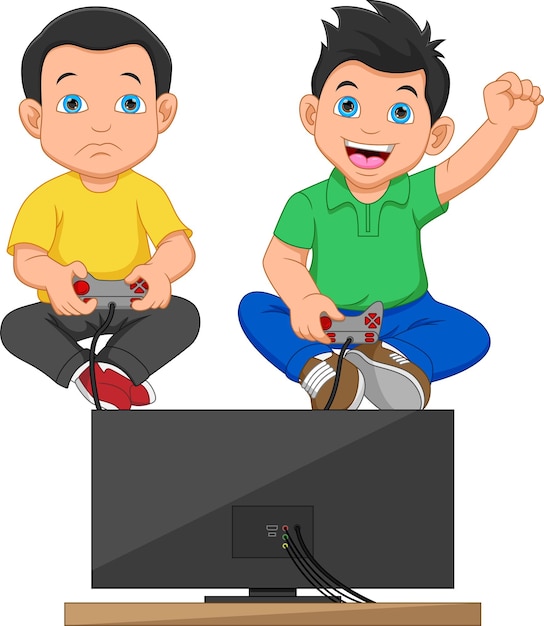The image is a clipart-style depiction of two young boys playing a video game, illustrated in a cartoon fashion against a pure white background. The scene focuses on the back of a black TV with three ports and several wires, sitting on a tan wooden table. Both boys are holding wired gaming controllers connected to the TV. On the left is a boy dressed in a yellow shirt, black pants, and red shoes. He has light skin, blue eyes, and short dark hair. His expression is sad, and he is sitting cross-legged. To the right, a similar-looking boy with light skin, blue eyes, and slightly longer styled dark hair is adorned in a green shirt, blue pants, and brown shoes. He appears jubilant, raising a fist in victory and smiling broadly, showing his front teeth and tongue. The contrasting emotions between the two boys are a central feature of this detailed clipart image.